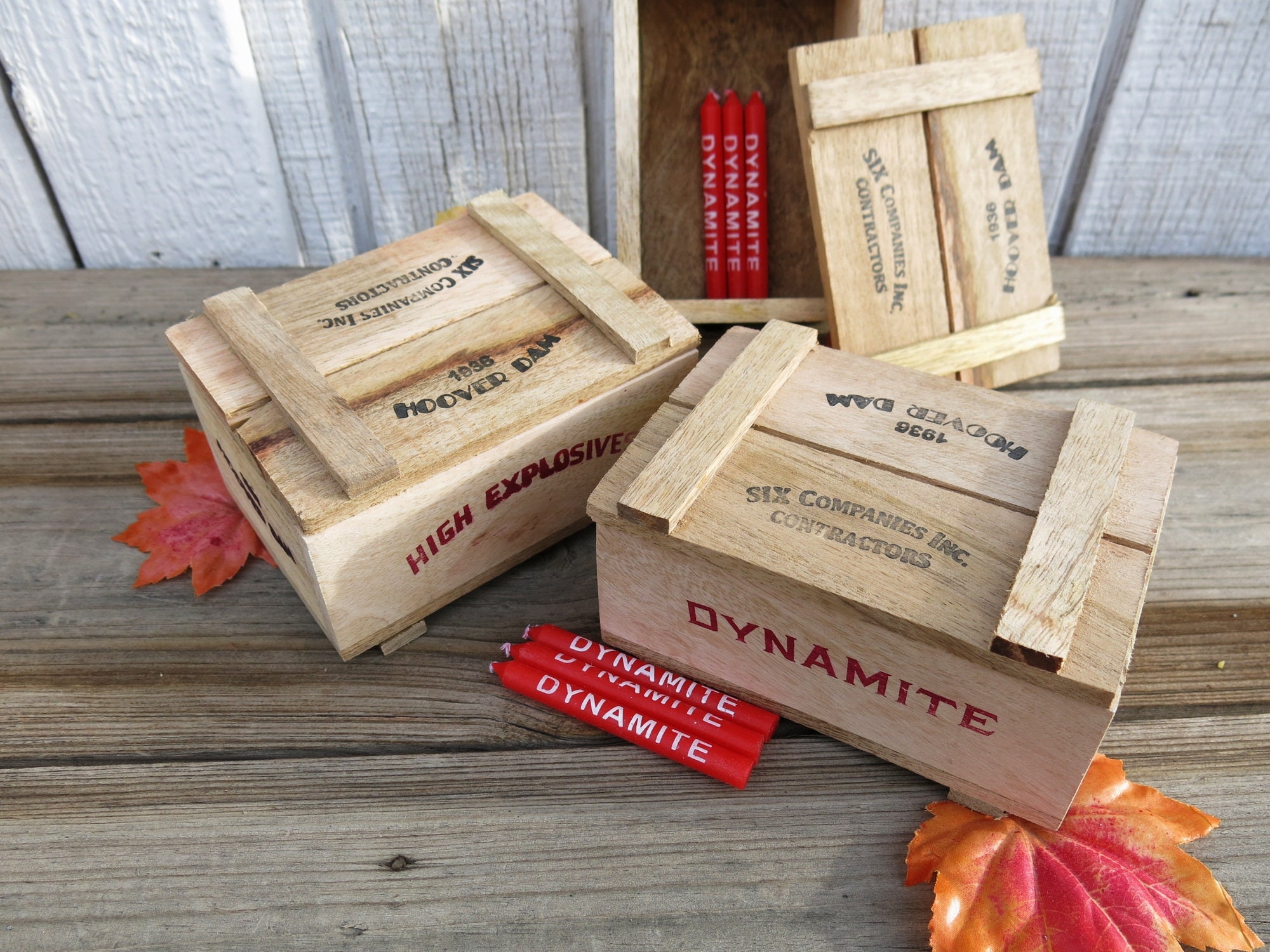The image depicts an outdoor scene during the daytime, featuring three light beige wooden boxes marked as "dynamite" and "high explosives" in bold red fonts. Each box also bears the inscriptions "1936 Hoover Dam" and "Six Companies Inc. Contractors" in black font. One of the boxes is open, revealing three red cylinder-shaped candles with white wicks, each labeled "DYNAMITE" in white capital letters. In front of these wooden boxes are the same red candles and a few strategically placed orange and red autumn leaves, enhancing the rustic wooden settings, including horizontal slats and a vertical wooden structure painted white, possibly a fence or wall.